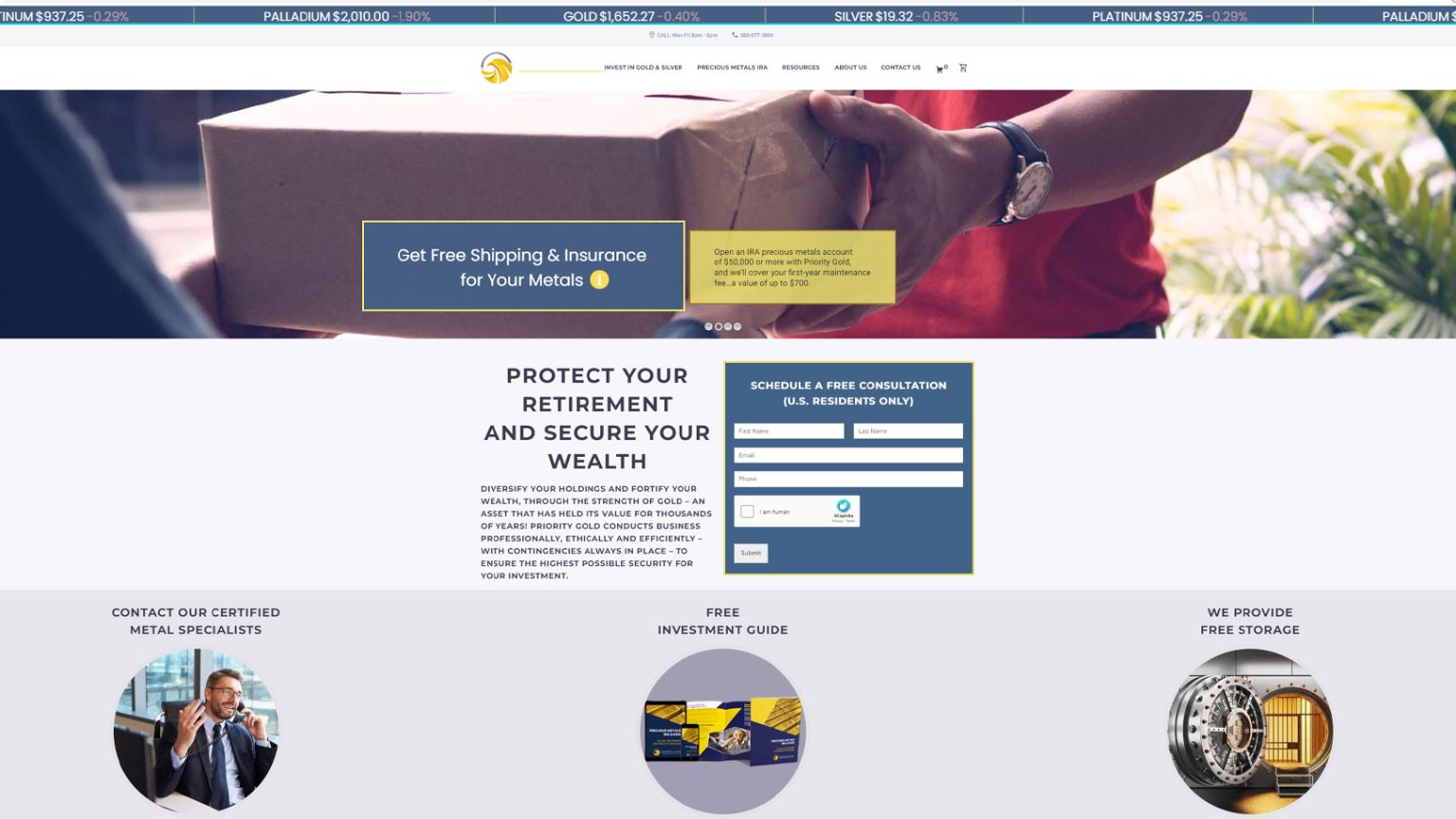The image appears to be a screenshot from a financial website with various sections and informational elements.

At the top of the page, a greenish-blue border runs across the screen, featuring essential market data. On the upper left, it displays "INUM, $937.25." Opposite that, on the right, it shows "Palladium, $2,010." Next to these, the prices of precious metals are listed: "Gold, $1,652.27," followed by "Silver, $1,932.00,” and finally, "Platinum, $937.25."

Dominating the middle section is an image of a person wearing a red t-shirt and a watch on their left hand, holding a box containing round paper items. This visual is accompanied by a call-to-action text: "Get shipping and insurance for your metals."

Below this image, a grey area provides additional information: "Protect your retirement and secure your wealth." Beneath this, a prominent blue square invites users to "Schedule a free consultation, U.S. residents only."

The bottom of the screen features another grey area containing three circular icons. The first icon is labeled "Contact our certified metals specialist," accompanied by an image of a male in a blue suit sitting at a desk, talking on the phone. The second shows what looks like a brochure, labeled "Free investment guide." The third icon, positioned on the far right, depicts a bank vault and states, "We provide free storage."